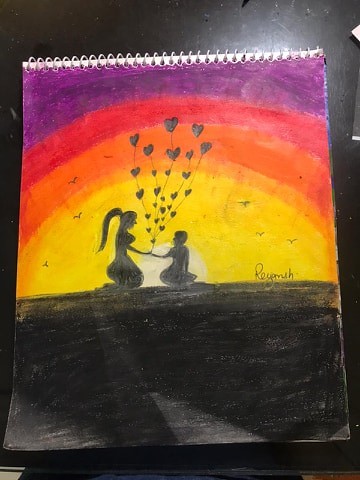This vertical photograph captures an intricate piece of art created in a spiral-bound sketchbook with silver spirals at the top. The entire sheet is vividly colored, showcasing a stunning sunset in the top half. The sunset transitions smoothly from yellow near the horizon line, through shades of orange and red, finally culminating in a rich purple towards the top. Against this vibrant backdrop, two black silhouettes are depicted sitting at the horizon line. A larger woman with a ponytail is holding hands with a smaller, kneeling figure who presents a bouquet of hearts reaching upwards towards the sky. The combined elements of color and intimate interaction create a poignant and visually arresting composition.